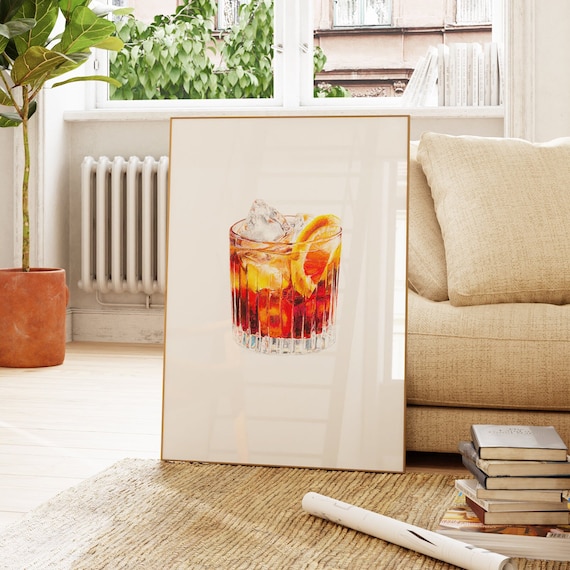The indoor daytime living room scene features a bright and somewhat cluttered space. Dominating the foreground is a close-up view of a painting propped against the side of a beige or cream-colored sofa with throw pillows. The painting depicts a glass filled with a brownish cocktail, ice cubes, and a slice of citrus fruit, likely a grapefruit or an orange. 

To the left of the sofa, a stack of around seven books rests on a light brown, thatch-style rug. A white tube lies on the floor in front of the books. The room features wooden flooring with horizontal lines and a beige carpet. The back left corner showcases a reddish clay pot holding a small tree or palm. 

There's a white wall adorned with a radiator and a shelf displaying a haphazard arrangement of white papers. The background reveals a window with a view of a neighboring building and greenery, hinting at the outdoor landscape beyond.